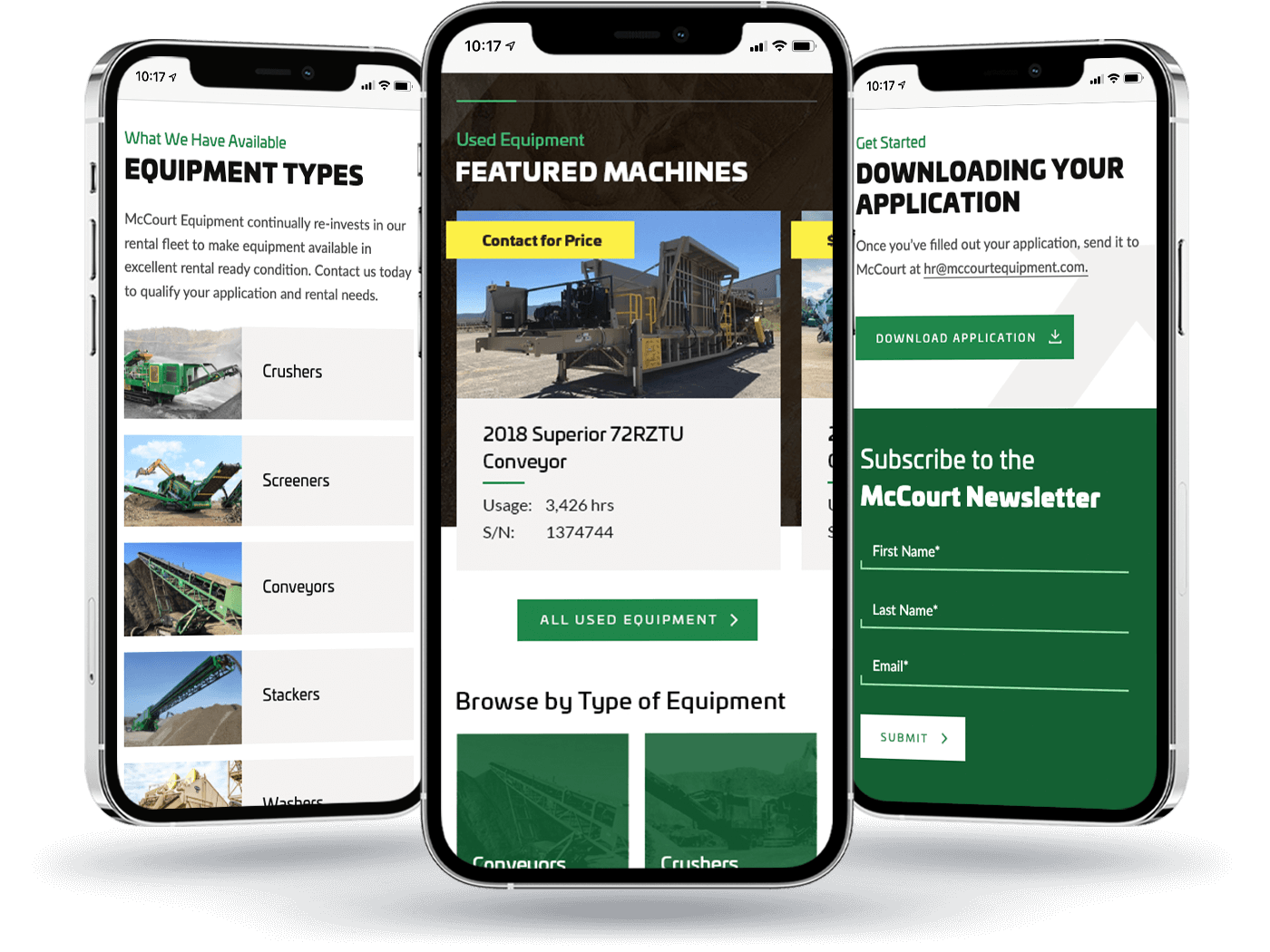The image showcases three smartphones, each displaying a different screen from a website, meticulously aligned with one in the center and the other two slightly behind it on either side. Every phone displays the same time and identical icons at the top of their screens. 

The central phone’s screen features a detailed listing for a 2018 Superior 72RZTU conveyor, under the headings "Used Equipment" and "Featured Machines". It includes specifications such as 3,426 hours of usage and a serial number of 1374744. 

The phone to the left highlights the range of equipment available from the company, listing categories such as crushers, screeners, conveyors, stackers, and washers. 

The phone on the right prompts users to start the application process by downloading a form and provides instructions to send the completed application to McCourt Equipment’s HR department via the email address hr@mccourtequipment.com. Additionally, it has a subscription section for the McCourt newsletter, requiring first name, last name, and email, followed by a submit button. 

This setup effectively showcases the company's diverse offerings and user-friendly application process.